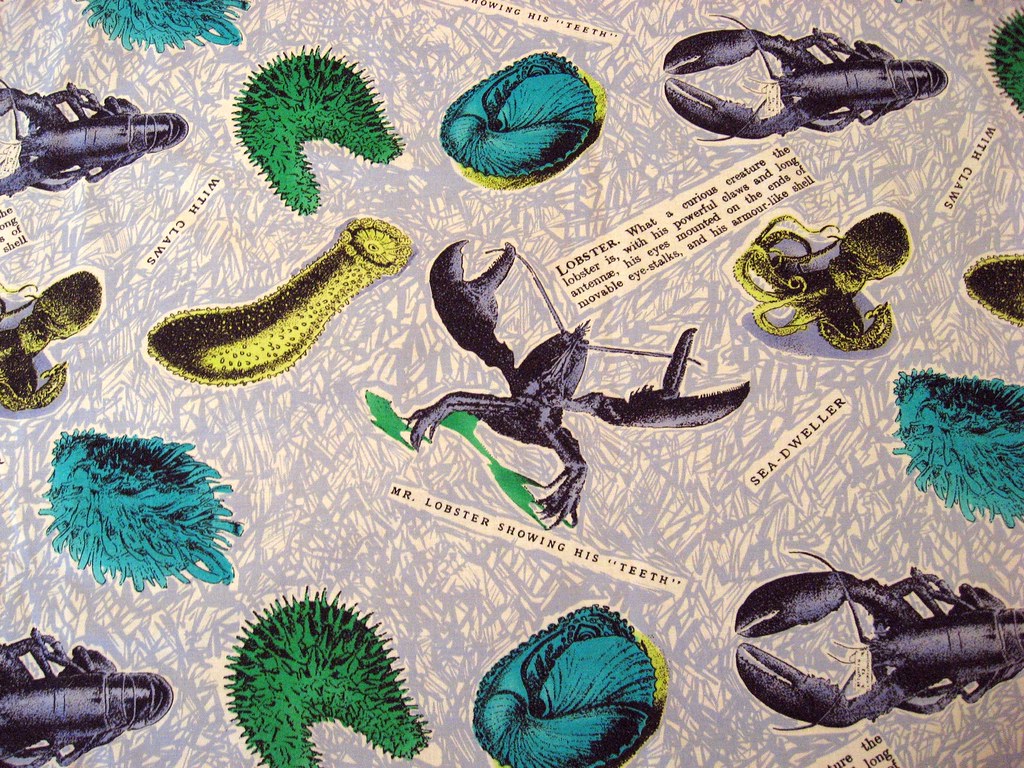This image appears to be either wrapping paper, the cover of a book, or a poster, featuring a vibrant underwater scene filled with various sea creatures. The backdrop is a blend of blue and cream hues, abstractly scribbled to add texture. Scattered across this background are assorted sea creatures illustrated in bright, captivating colors. Among them are a bluish-gray lobster with detailed shading, an octopus displaying a yellow underside and a black top, bright green sea sponges, and teal sea urchins with a hint of yellowish green.

Interspersed among the sea creatures are pieces of what seem to be newspaper or dictionary clippings. These fragments carry quirky descriptions and labels, such as "Mr. Lobster showing his teeth" and "Sea Dweller." One clipping above the lobster provides a detailed description: "Lobster, what a curious creature the lobster is, with his powerful claws and long antennae, his eyes mounted on the ends of movable eye stalks, and his armor-like shell." The notes are written in black typewriter-style letters.

Purple lines accentuate the tan-colored background, providing additional depth. The overall scene looks animated, with graphic elements that create a lively and whimsical underwater tableau. The combination of detailed illustrations and textual annotations scattered around enhances the visual interest, making it a rich and engaging image.